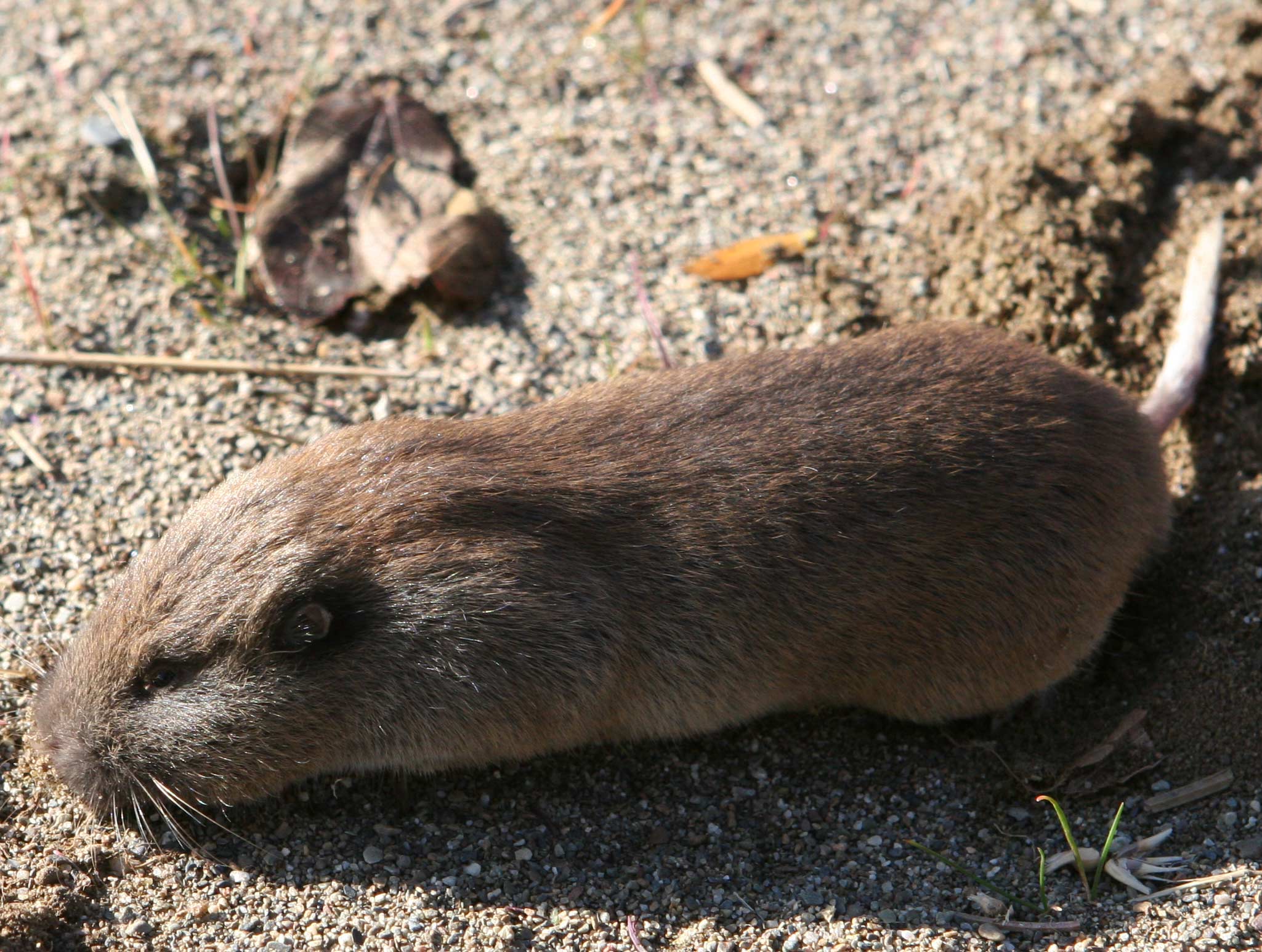This close-up photograph captures a small rodent, likely a mouse or rat, with a brown body and a long, slender tail that is notably white. The animal's fur is brown, and it features distinct whiskers and small ears. This rodent is pictured lying on a ground surface that comprises dirt mixed with small rocks, sand, and pebbles, likely an outdoor setting. The scene also includes dried brown leaves, small twigs, and possibly some dead reeds scattered around. The image, oriented as a horizontal rectangle, appears to be taken from a slightly elevated angle, looking down. The animal is oriented with its nose pointing to the left and its tail curving towards the top right. The sunlight comes from the left, casting a shadow of the rodent in the foreground, indicating that it is daytime. Aside from the primary subject, a tiny plant bud is visible in the bottom right corner, poised to grow amidst the scattered ground debris.